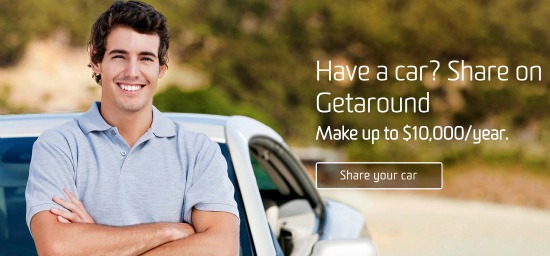This advertisement for the business "GetAround" features a vibrant, landscape-oriented photo showcasing a young Caucasian man in his 20s. He has short, dark hair and is dressed in a light gray, short-sleeved collared polo shirt. The man stands confidently with his arms crossed, leaning against a pristine white car behind him. His expression is joyful, highlighted by his smile and eyes crinkled into half-moon crescents, suggesting he might have dark-colored eyes.

The scene is set in broad daylight on a serene country road, with out-of-focus trees and greenery adding a peaceful, natural backdrop. On the right side of the image, bold white text reads, "Have a car? Share on GetAround. Make up to $10,000 per year." Below this message, a call-to-action button outlined in a white rectangle prompts viewers with the text, "Share your car." This advertisement effectively combines a compelling visual narrative with clear, enticing information about the benefits of using the GetAround service.